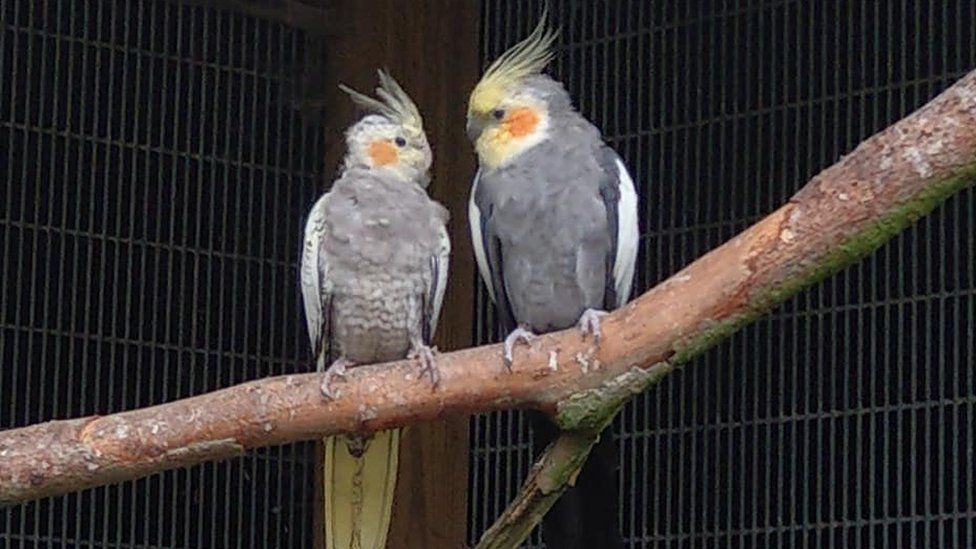This is a horizontal rectangular photograph depicting two cockatiels perched inside a cage, characterized by closely spaced, dark gray or black bars. Both birds are situated on a diagonal tree branch that extends from the upper right to the lower left of the image. The background consists of dark vertical stripes.

The cockatiel on the left features a lighter gray chest, a pale yellow head with distinct individual feathers forming a crest, and an orange circular patch on its cheek. It has a yellow tail with less pronounced black markings.

The cockatiel on the right, slightly larger in size, has a darker gray chest, a more vivid yellow head, and an equally pronounced orange cheek patch. Its tail exhibits darker coloration, including black areas underneath.

Both birds have black eyes and are gazing at each other. Their light gray claws grasp the thick tree branch, which is broad enough to prevent their claws from fully encircling it. Overall, the cockatiels' shared traits of gray chests, orange cheek patches, and spiked feather crests make them visually and behaviorally engrossing.